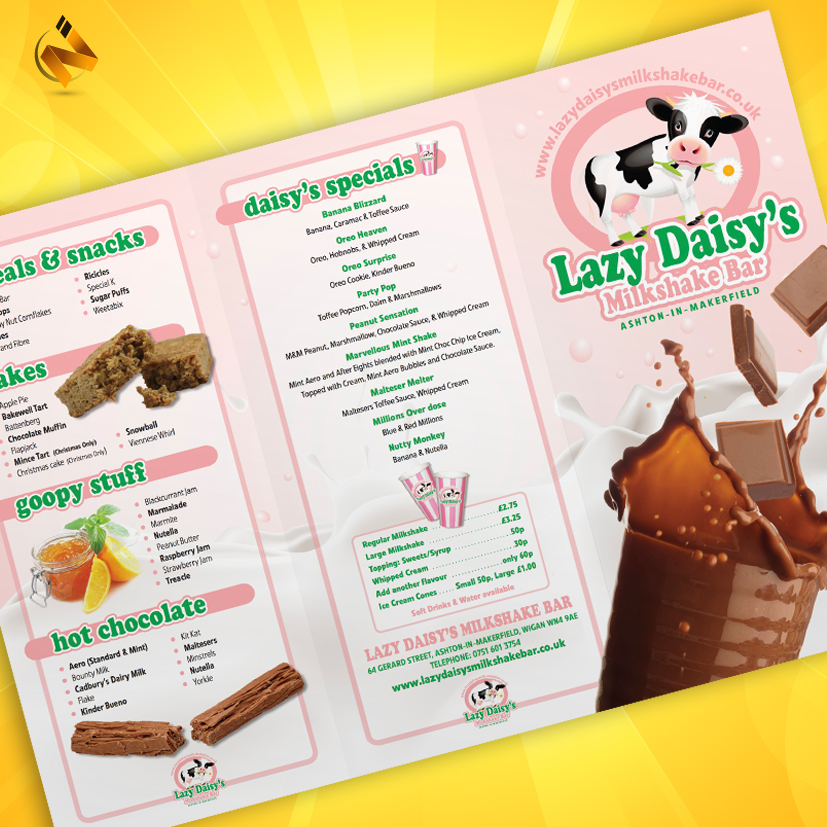In this colorful image, the focal point is a centrally placed menu from "Lazy Daisy's Milkshake Bar" at Ashton Inn, Makerfield. The menu boasts a vibrant design with a main pink background and a cheerful multi-colored yellow backdrop. The bottom portion depicts a milk splash motif, effectively drawing attention to the delicious offerings. The menu is split into three sections: 

- The left section titled "Meals and Snacks" lists Special K, Sugar Puffs, Weetabix, Apple Pie, Bakewell Tart, and Chocolate Muffin. It continues with "Goopy Stuff" featuring different jams, followed by an assortment of "Hot Chocolate" options including Aero Bars, Kit Kat, and Maltesers.
  
- The middle section showcases "Daisy's Specials" with items like Banana Blizzard, Oreo Surprise, Party Pop, Peanut Sensation, Marvelous Mint Shake, Malt Caesar, Malt Sur, and Millions Over Dose.
  
- The rightmost part of the menu includes an endearing cartoon image of a cow holding a daisy in its mouth, perfectly encapsulating the playful essence of the establishment. Here, the header "Lazy Daisies" is prominently written in green, with "Milkshake Bar" featured in pink beneath it.

Additionally, the top left corner of the image displays a logo further emphasizing the branding. The menu is illustrated with enticing images of a chocolate bar, various fruits, and a milkshake, inviting patrons to indulge in a delightful experience. The diverse color palette incorporates shades of yellow, orange, black, brown, pink, and green, enhancing the lively and welcoming atmosphere typical of a whimsical milkshake bar.